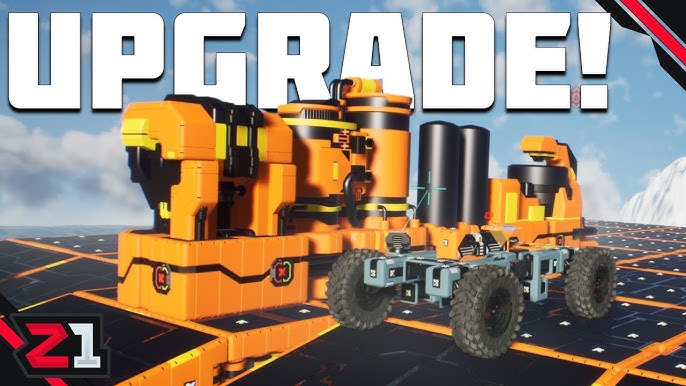The image in question appears to be a cover for an online game, prominently featuring the word "Upgrade!" in bold white letters at the top, and the letters "Z1" in the lower left corner. The scene is computer-generated, likely representing a setting where upgrades and efficiency improvements are a focal point. At the center of the image, there's a large machinery unit or building that features a mix of yellow and black colors, including crates and storage containers, some with lids that seem to open. Adjacent to this building is a small vehicle, which appears to be some form of tractor or transport car, characterized by its four black tires, a yellow top, and two cylindrical tubes protruding from it. The vehicle moves along a pathway comprised of black squares, possibly hinting at a factory floor or an industrial conveyor system. The background showcases a blue sky with clouds, giving the scene a somewhat open and expansive industrial environment. The black ramp with orange grid lines under the machinery further emphasizes the setting's industrial theme.